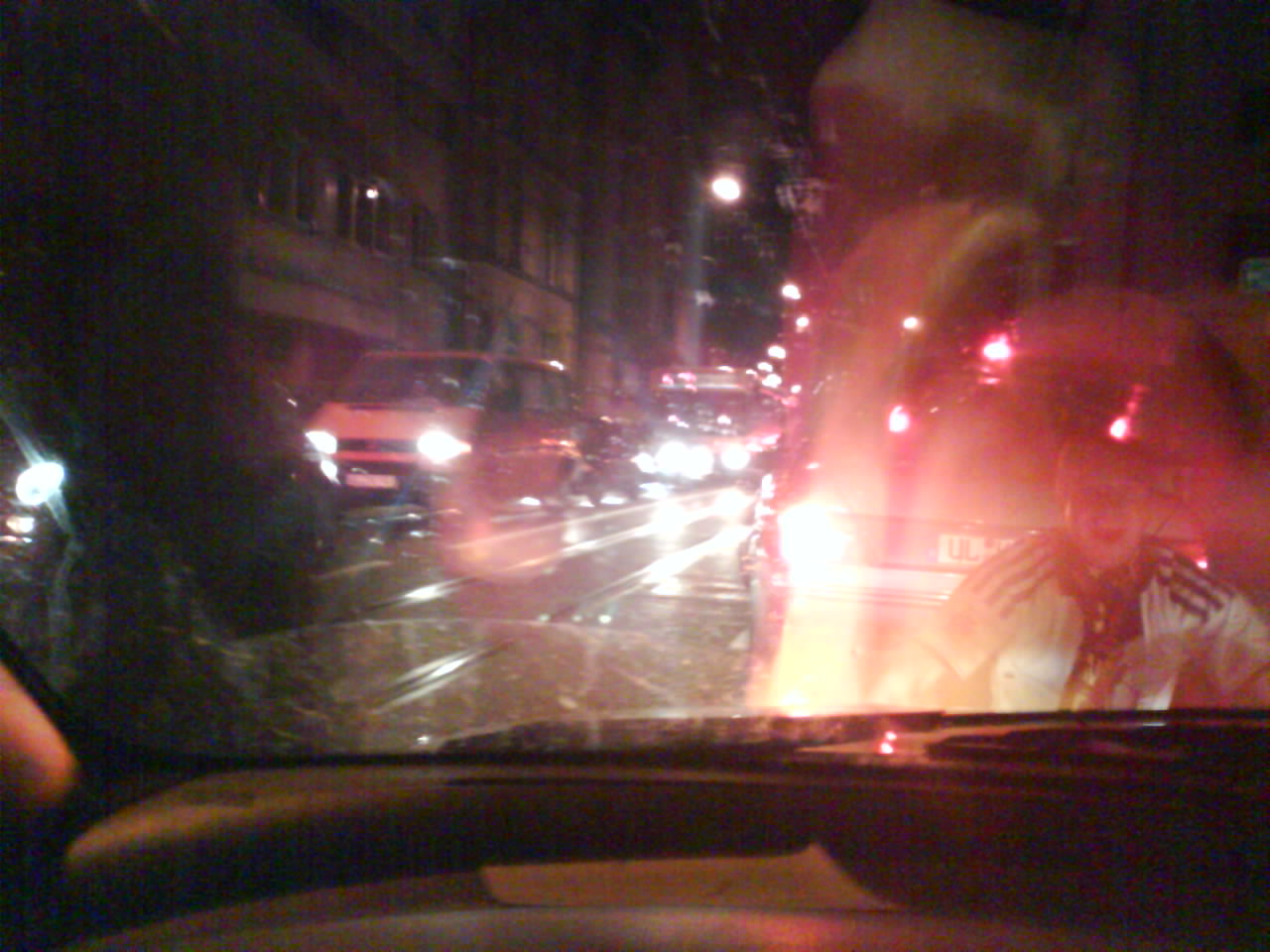This nighttime photograph, taken from the inside of a car, presents a blurry and chaotic scene due to a combination of factors such as a dirty window, reflections, and possibly rain. The dashboard, which is black, is partially visible. There’s also a glimpse of someone's index finger and possibly their hand obstructing part of the camera lens. 

In the foreground, a person wearing a white shirt with black stripes near the shoulders stands in front of the car. They have their mouth open in a surprised expression. Beyond this person, a car with illuminated brake lights can be seen, part of its license plate displaying the letters 'U' and 'L'. 

Further details reveal vehicles with smeared, orangey-red tail lights and white headlights from oncoming traffic. Among these, a white van and a bus are visible. The scene is set against a backdrop of large buildings and streetlights on both sides of the road, under a wet or rainy night sky, accentuating the reflections and blurs. Overall, the image captures a moment of confusion through a conflagration of reflection, dirt, and car window distortions.